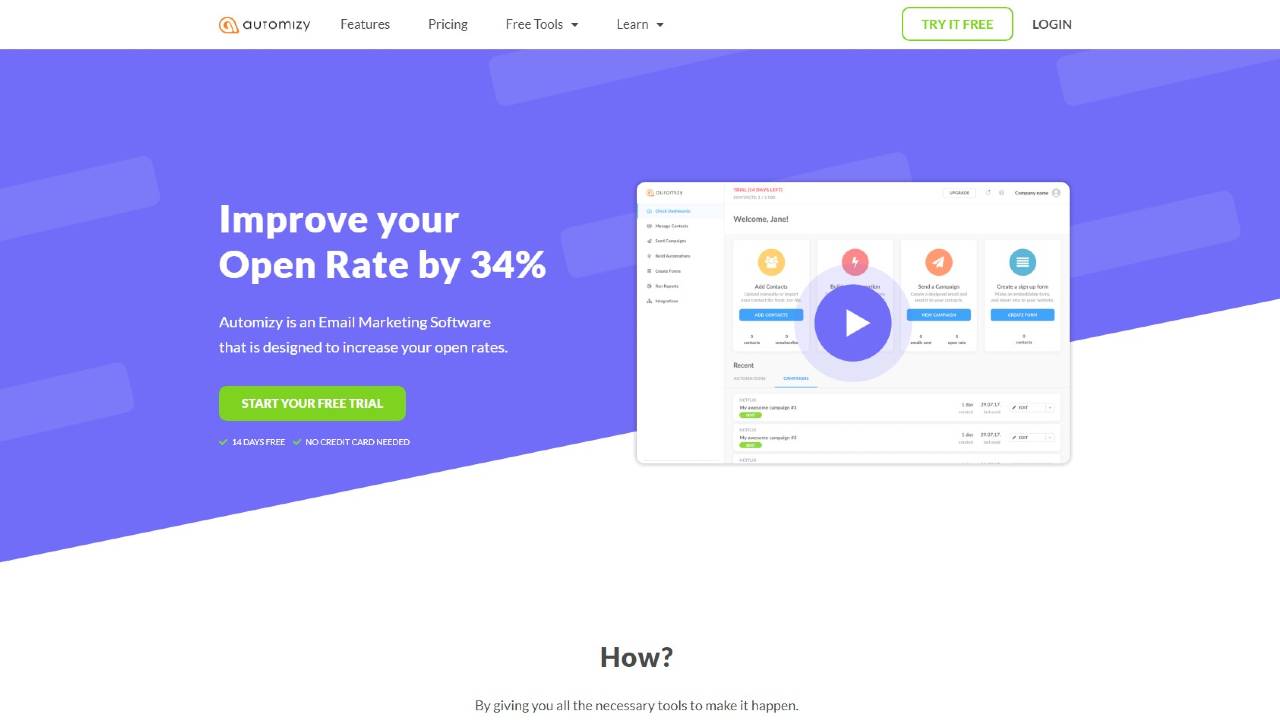Here's the cleaned-up and detailed descriptive caption:

---

This image depicts a website homepage for Automizee, an email marketing software aimed at improving open rates. At the top, the navigation menu features options labeled "Features," "Pricing," "Free Tools," and "Learn," along with buttons for "Try it Free" and "Log In." The background is a light blue, creating a calming and professional aesthetic. Prominently displayed in the center, a bold statement reads, "Improve your open rate by 34%." 

Below this headline, there is a brief description: "Automizee is an email marketing software designed to increase your open rates." 

Immediately underneath, a green call-to-action button invites users to "Start your free trial," specifying that the trial lasts for 14 days and does not require a credit card.

To the right of this button, there's a small play icon suggesting the presence of a video, although the details of the content are not discernible due to small lettering.

At the bottom section, in bold black letters, the word "How" is followed by a statement in smaller font: "By giving you all the necessary tools to make it happen."

---

This caption provides a thorough description of the website's visual and textual elements, ensuring clarity and completeness.